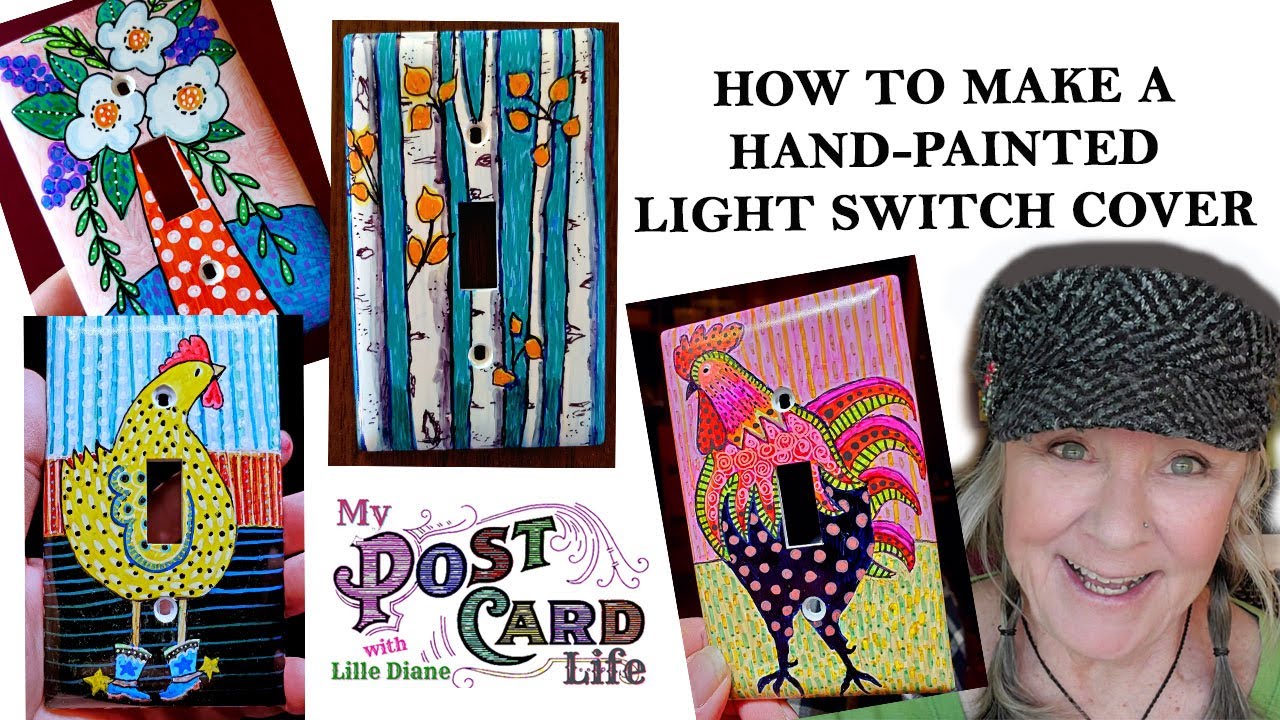The image is an instructional guide on how to make a hand-painted light switch cover, with the text prominently displayed at the top right. In the bottom right corner, there is an old woman with a smiling face; she has blonde hair in two braids tied with black ponytail holders and is wearing a gray hat with stripes and a bill, a black necklace, and a green shirt. She holds up one of the hand-painted light switch covers, which features a pink rooster with polka-dotted legs, a striped body, and swirly designs. To her left, there are four additional light switch covers: another yellow rooster, one with a red vase filled with white and purple flowers and green leaves, one adorned with blue vertical stripes and flowers, and another with a rooster that has pink and black sections and polka dots at the bottom. The text at the bottom of the image reads, "My postcard life with Lily Diane."